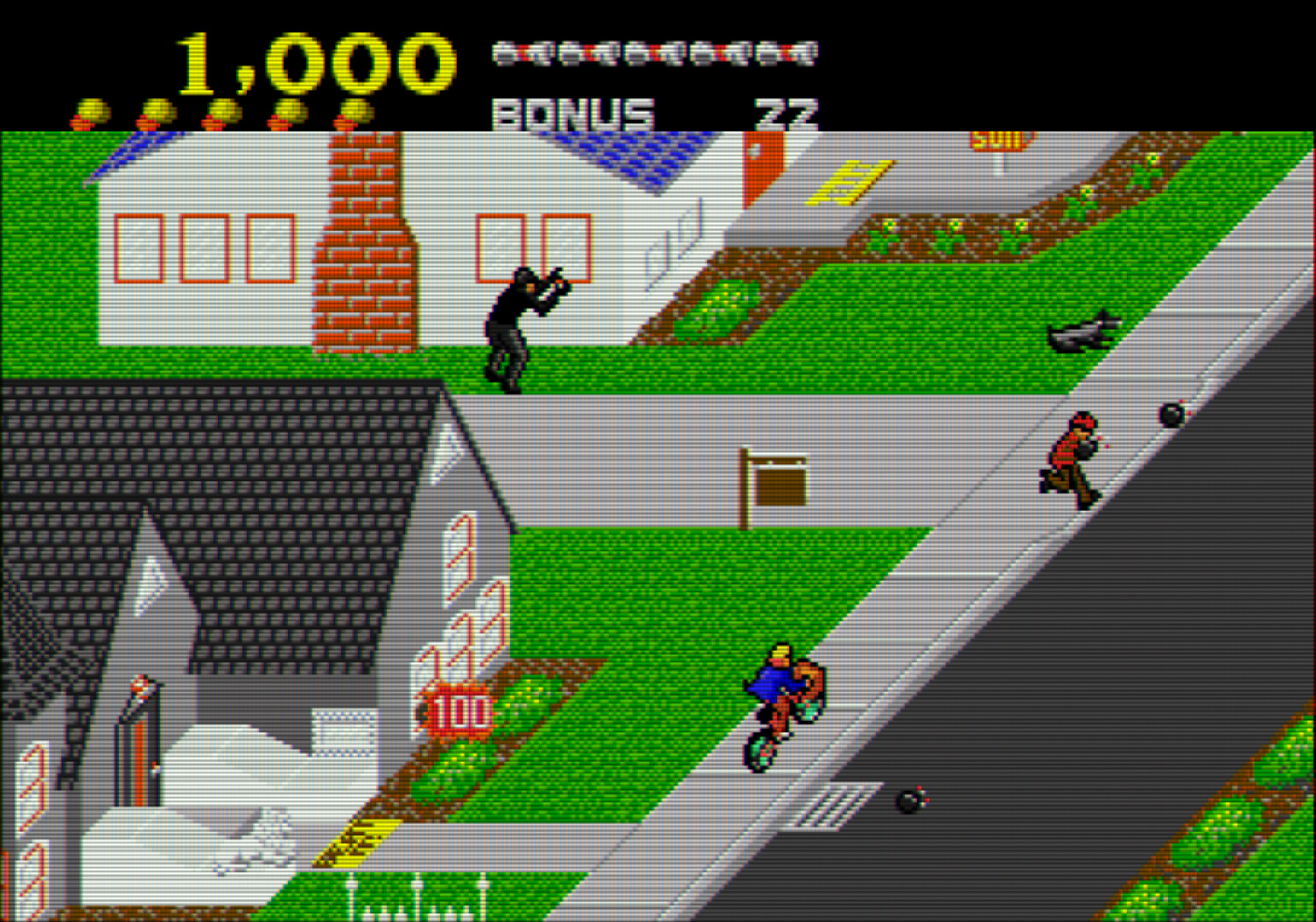A pixelated screenshot from an old-school video game, depicting a quaint, suburban neighborhood scene. The environment features three gray homes with white windows and a distinctive white house with a purple roof and chimney, set against an old-fashioned backdrop of low-resolution graphics dominated by whites, grays, and greens. A character in blue attire is riding a bike on the sidewalk, while another person is poised to cross into the street. Various elements on the screen suggest gameplay metrics, including a score indicated by "1000" at the top, "bonus 22," and a "100" superimposed over one of the houses. The scene appears to capture the essence of a charming, retro gaming neighborhood, with hints of point-based objectives scattered throughout.